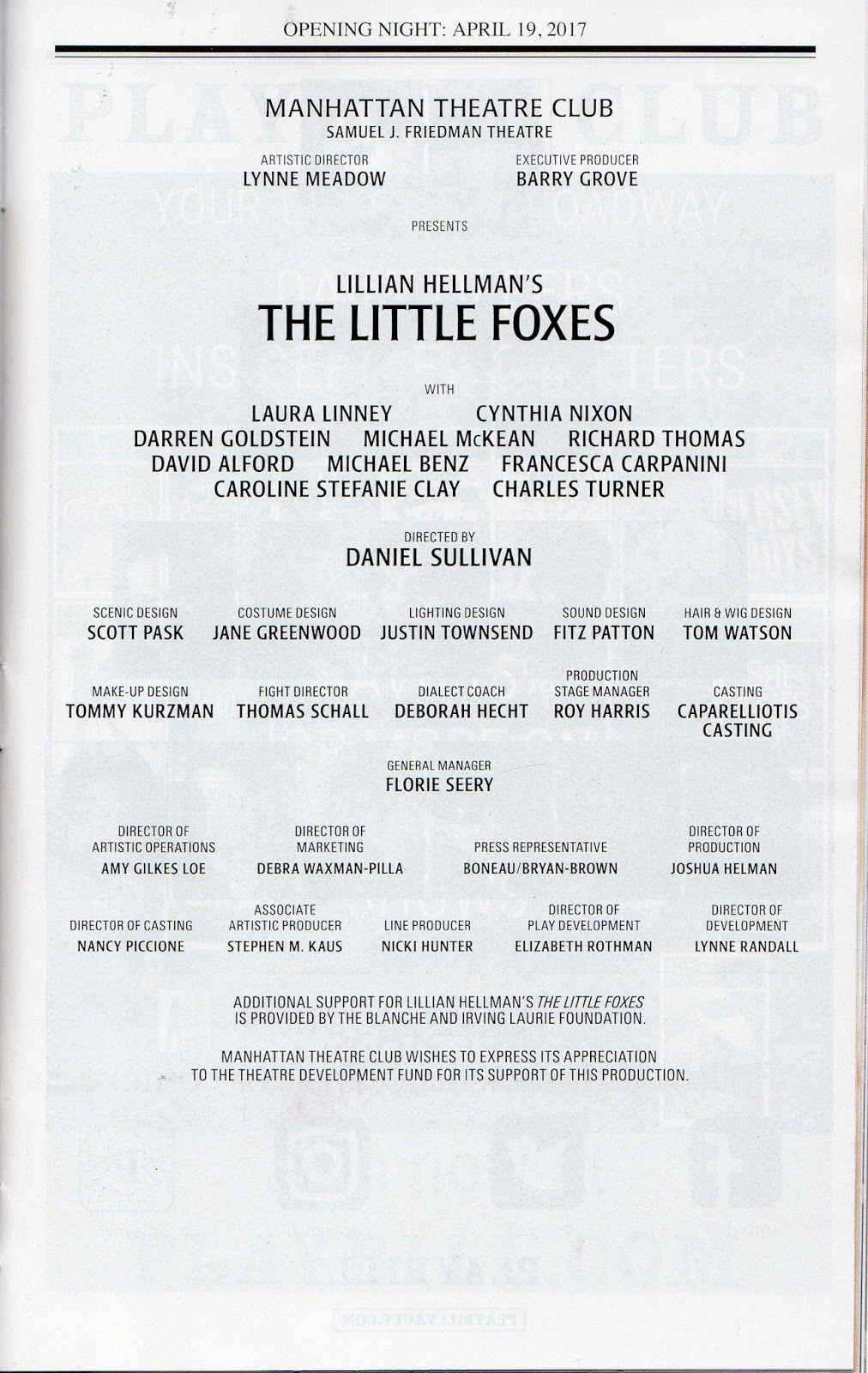This image is a scanned page from a playbill for the opening night of "The Little Foxes," a play by Lillian Hellman, held at the Manhattan Theatre Club's Samuel J. Friedman Theatre on April 19, 2017. The rectangular poster features prominently legible black capital letters on a white background with some bleed-through text visible from the reverse side. The top portion reads "Opening Night April 19, 2017," followed by a horizontal black line. Below the line, the text mentions "Manhattan Theatre Club," "Samuel J. Friedman Theatre," "Artistic Director: Lynn Meadow," and "Executive Producer: Barry Grove." The subsequent lines, in larger font, announce the play "Lillian Hellman's The Little Foxes," starring Laura Linney, Cynthia Nixon, Darren Goldstein, Michael McKean, Richard Thomas, David Alford, Michael Benz, Francesca Carpinini, Carolyn Stephanie Clay, and Charles Turner. The play is directed by Daniel Sullivan. Additional credits for scenic design, costume design, lighting design, and other contributions follow, though the smaller font sizes render these details harder to read. The bottom of the poster contains a sizeable blank area, and the background is a light blue.